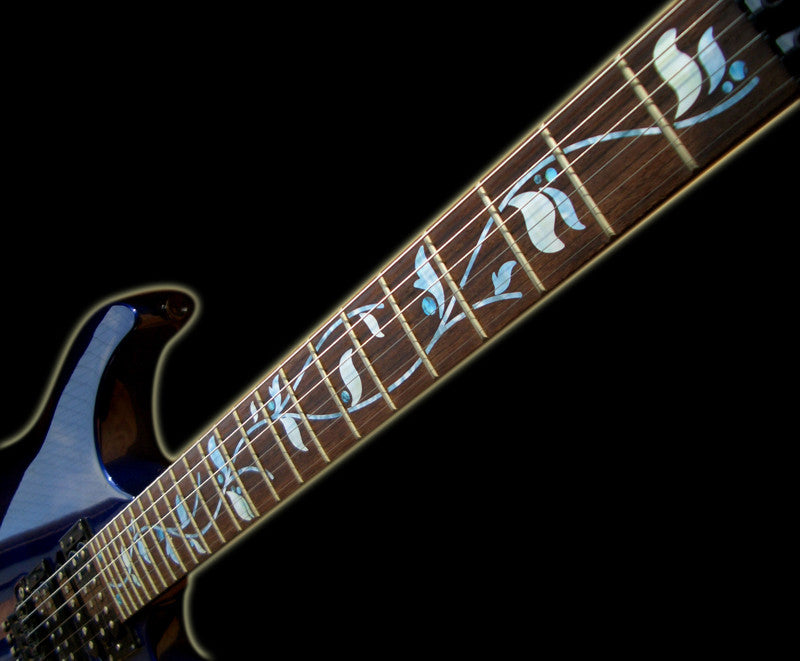This digital photograph features a close-up of a six-string electric guitar against a black background, capturing mainly the section where the body meets the neck. The guitar's body is crafted from a rich brown wood, and its bridge shares this brown hue. The neck of the guitar, however, steals the spotlight due to an exquisite inlaid abalone shell design depicted as a delicate vine with leaves. This intricate vine winds its way up the neck, transitioning from a light blue to turquoise, and gradually shifting to white at the top. The vine's stunning colors and craftsmanship suggest it is hand-done, adding a unique and visually arresting element to the guitar. The silver horizontal rungs (frets) span the length of the neck, harmonizing with the vine pattern and enhancing the overall aesthetic of the instrument.